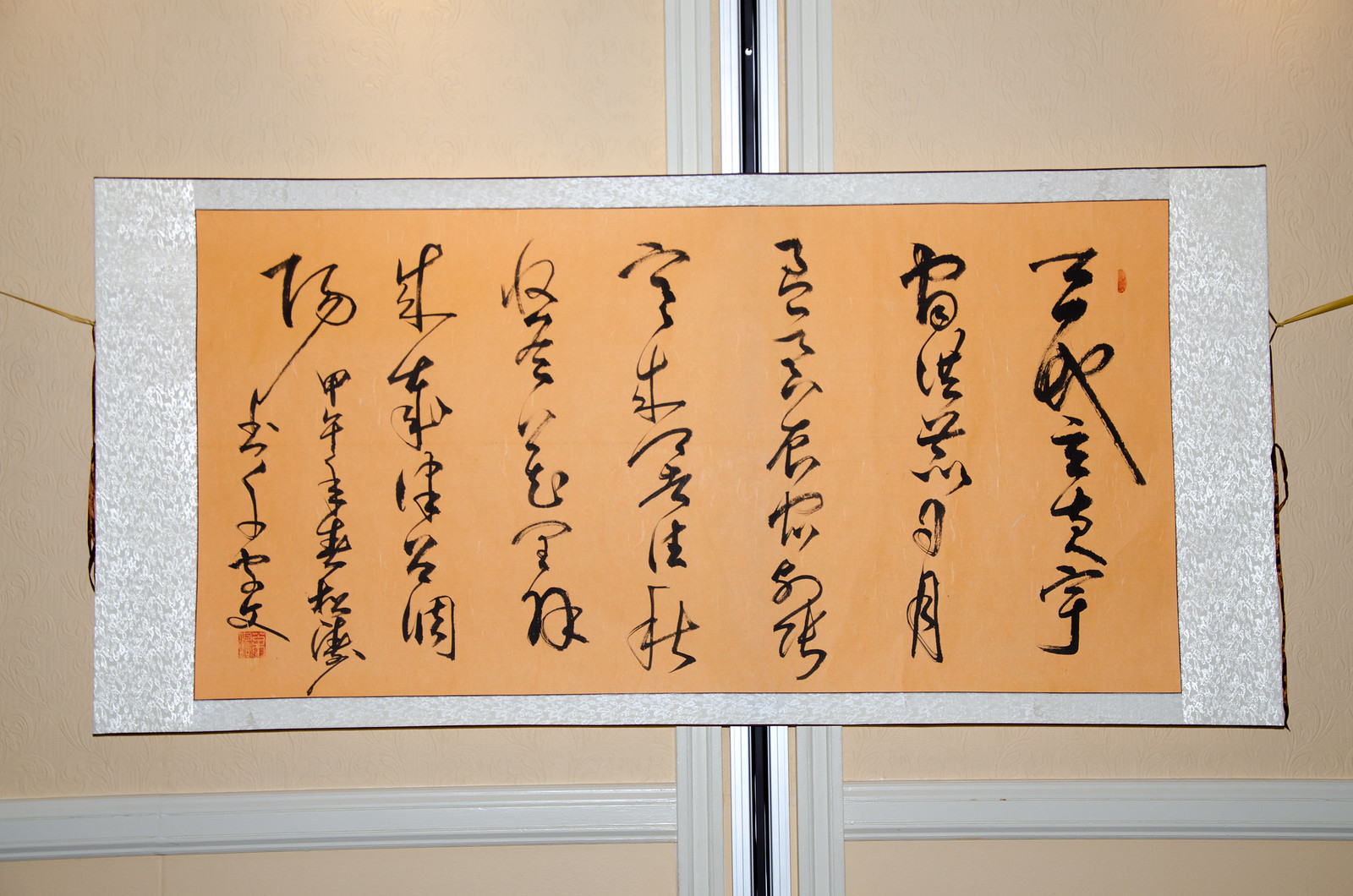The image captures an indoor scene featuring a detailed composition with a beige background. A piece of shimmering silver paper, its left and right edges gleaming subtly, is placed as the backdrop. On top of this glistening foundation lies an orange piece of paper, adorned with vertically-aligned black script. Additional visual interest is provided by an orange symbol, intricately stamped onto the bottom left corner of the orange paper, adding a touch of artistic flair to the meticulous arrangement.